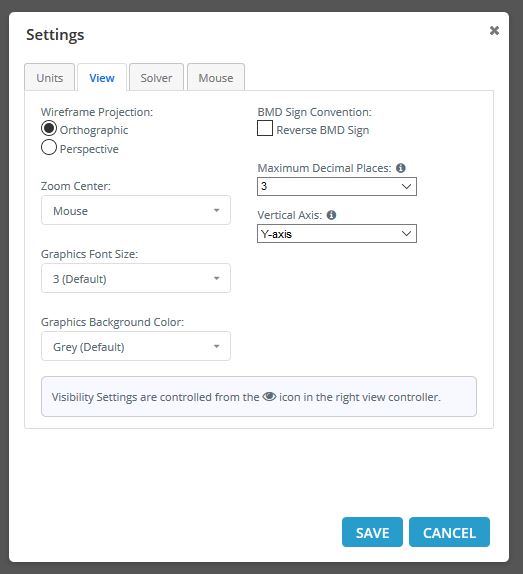This image shows a detailed view of a settings interface from a website. The settings box is white and floating against a dark gray background. At the top right of the settings box, there is a dark gray "X" button for closing the window. The top left corner is labeled "Settings."

Within the settings box, there are four menu options: "Units," "View," "Solver," and "Mouse." The "View" option is currently selected, indicated by its blue background, while the others remain dark gray.

Under the "View" menu, various settings are visible. The first setting is labeled "Wireframe Projection," featuring two options: "Orthographic" and "Perspective." The "Orthographic" option is currently selected, as indicated by a black circle next to it.

Following this, the "Zoom Center" setting offers a drop-down menu, from which "Mouse" is selected. Under "Graphics," the "Font Size" is set to "3 (default)" via a drop-down menu. The "Background Color" of the graphics is also configured through a drop-down menu, with "Gray (default)" selected.

Further down, it mentions that "Accessibility settings are controlled from the eye icon in the right view controller."

On the right side of the settings box, there is a section titled "BMD Sign Convention." There is an empty checkbox labeled "Reverse BMD Sign" next to it. Below this, it says "Maximum Decimal Places," accompanied by an information icon and a drop-down menu set to "3."

The next section is titled "Vertical Axis," with a drop-down menu selecting the "Y-axis." Finally, at the bottom right corner of the settings box, there are two buttons: a "Save" button with blue background and white font, and a "Cancel" button with the same blue and white color scheme.